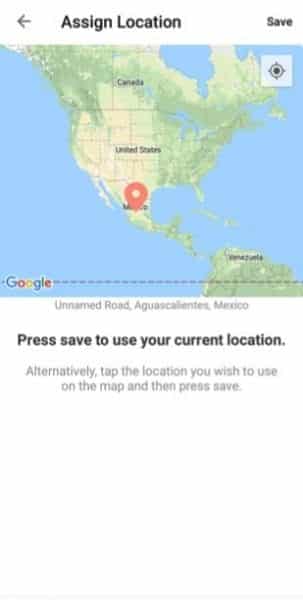A Google Maps screenshot depicts a zoomed-out view of North America, extending to parts of Central America and the northern region of South America, including Venezuela and a portion of Brazil. The map features a marker placed in Aguascalientes, Mexico, named "Unnamed Road." An instruction overlay at the bottom of the screen prompts users to "Press save to use your current location, alternatively tap the location you wish to use on the map and then press save." The map also highlights topographical differences, showing the Midwest of the United States as notably flat and the eastern regions as more elevated. Similarly, the northern part of Mexico displays varied elevation. Color coding on the map indicates terrain types: green for mountainous and high-elevation areas, and a yellowish hue for lower elevations.